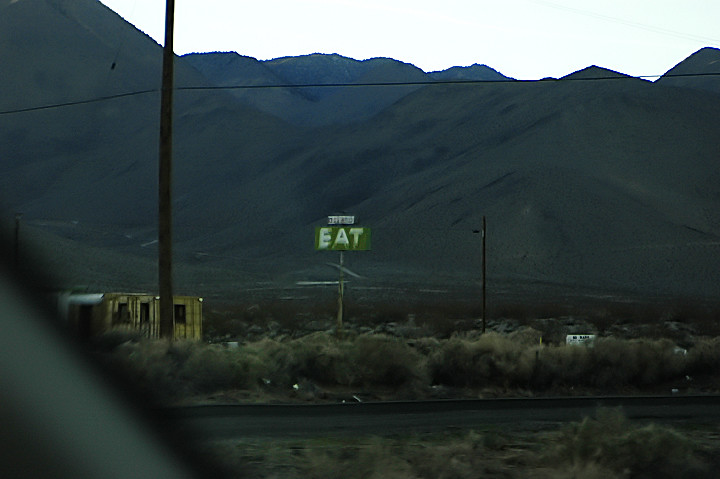This slightly blurry photograph captures a bleak, outdoor scene during daytime, evoking a dystopian atmosphere. A degraded yellow mobile home with an aluminum-colored roof and three visible windows stands to the left, projecting a sense of neglect. Adjacent to it, a tall, light-colored telephone pole with a single wire stretches across the image, emphasizing the desolation. Dominating the center is a green, rectangular sign mounted on a wooden pole, with the large, white capital letters spelling "EAT," partially worn away, suggesting decay. The scene includes a small white building in the distance, lower right, along a road flanked by dry grass, low brush, and weeds, indicating a possibly western U.S. location. Further adding to the isolation, a partial view of train tracks is visible, hinting at forgotten journeys. In the background, a vast mountain range with tree-covered ridges under a nearly white, overcast sky, completes this grim, grainy tableau of abandonment.